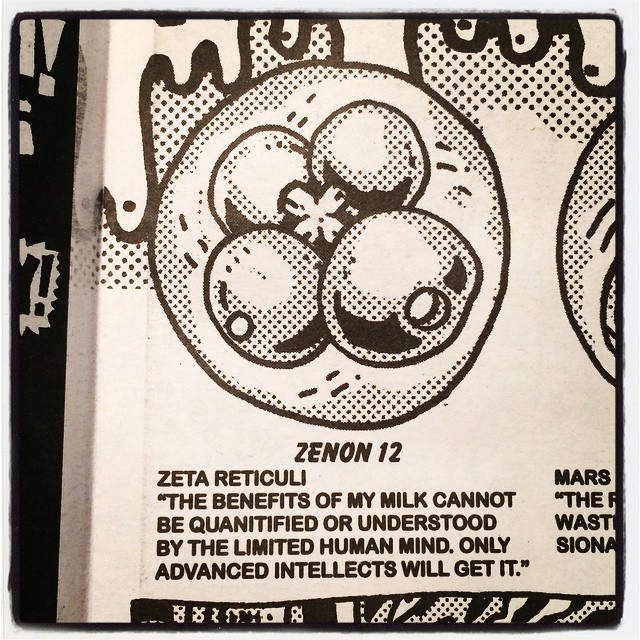The image depicts a detailed, printed document on a white background. Dominating the upper portion is a black-and-white illustration contained within a circular border, featuring what appear to be blueberries or berries, rendered with dot work reminiscent of comic book shading. The berries are surrounded by decorative elements, including another partial circle with similar fruit on the upper right and a black band running down the left-hand side, adorned with gray text, decorative symbols, and an exclamation mark. Beneath the illustration, bold text reads "Xenon-12," followed by smaller text that states: "Zeta Reticuli. The benefits of my milk cannot be quantified or understood by the limited human mind. Only advanced intellects will get it." Additional text at the bottom right, albeit partially cut off, includes the words "Mars" and "the waste." The intricate design and cryptic wording suggest it might be a page from a comic book or an educational pamphlet targeted at readers with advanced knowledge or intelligence.